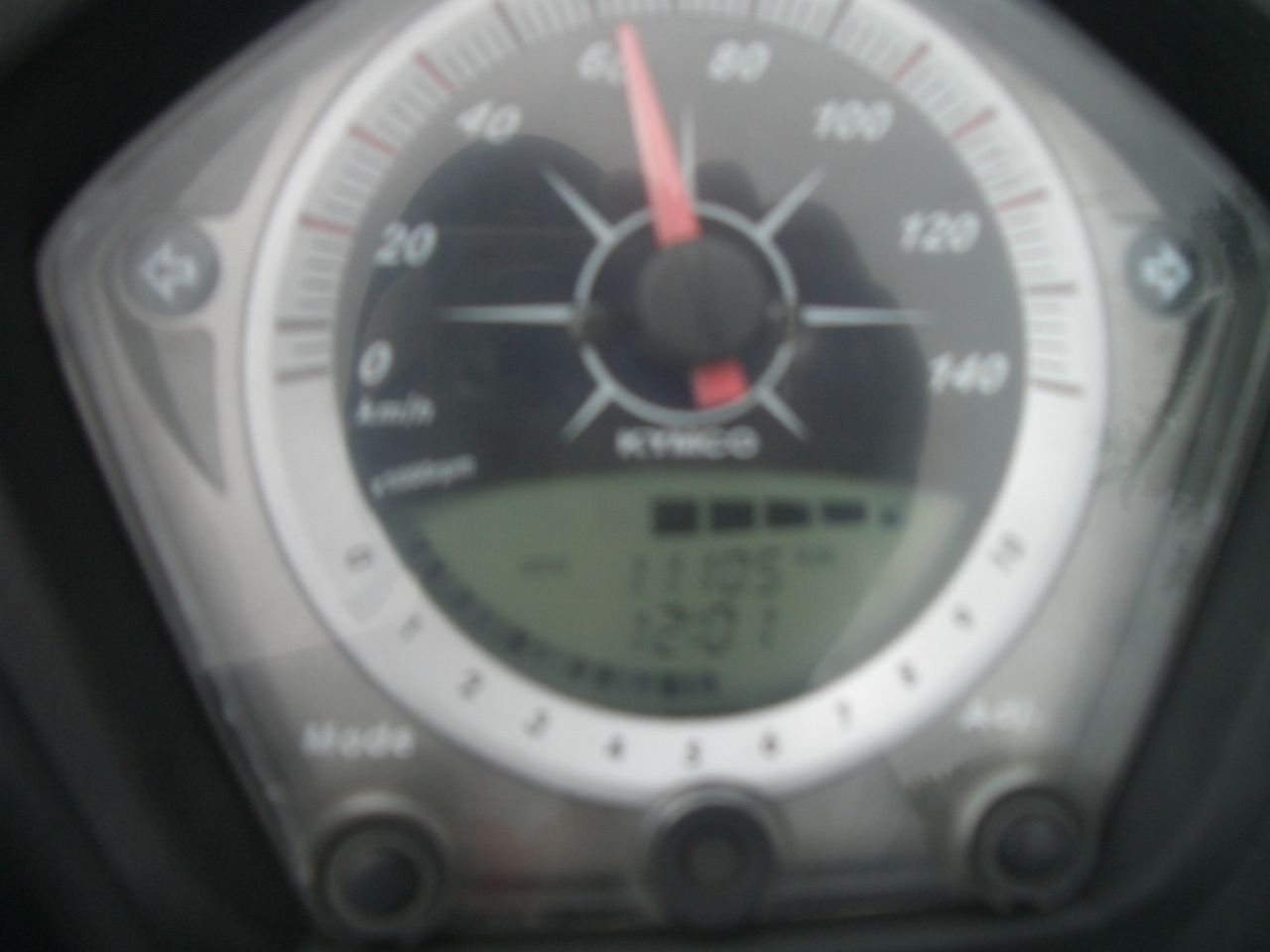An extreme close-up of a car speedometer is captured in intricate detail. The speedometer is prominently centered in the image, presenting a clear and precise view of its structure and markings. The background surrounding the central part is mainly black in the upper left and upper right quadrants, while transitioning to a dark gray hue below on both the left and right sides.

Framing the speedometer is a silver circle, which adds a touch of elegance and clarity. Immediately inside the left and right edges of this circle are two small gray buttons, each marked with a white arrow; the left button points left and the right button points right. 

At the outermost edge on the left side, a red line emerges, arching gracefully in a clockwise direction and marking various intervals along the way with an array of red and smaller black lines. This red line progresses through marked speed increments: 0, 20, 40, 60, 80, 100, 120, and 140 miles per hour, arranged around the dial.

Within this outer framework exists another inner black circle that houses a vibrant red needle. This needle stretches upward, pointing precisely to about 64 miles per hour. Below this needle, a small screen displays crucial information like the current time and the total mileage traveled.